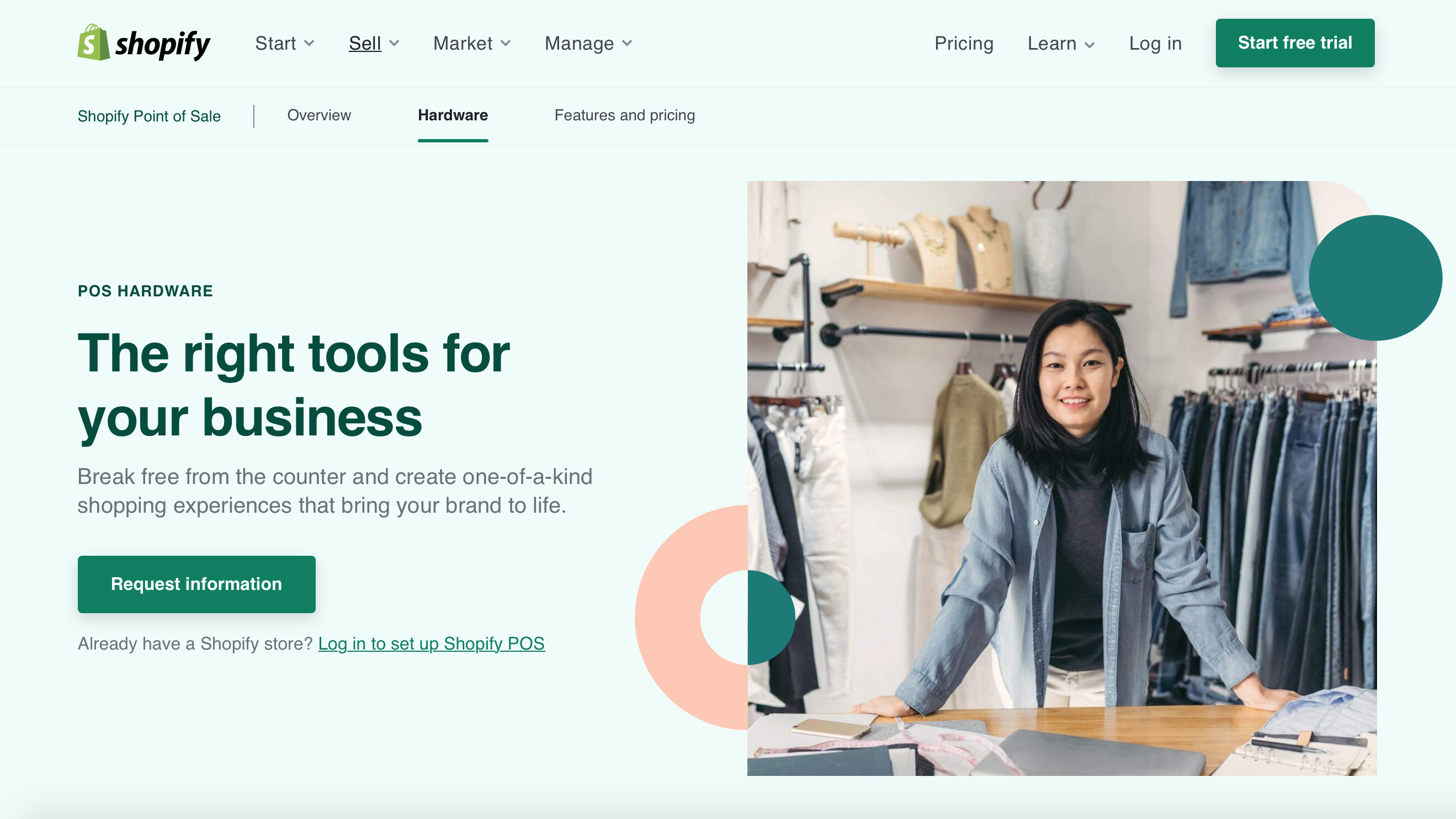Here's a detailed and cleaned-up caption for the image:

**Screenshot of a Shopify page in portrait mode:**

The background of the page is a light green color, providing a fresh and modern look. In the upper left-hand corner, the Shopify logo is prominently displayed. Directly next to the logo, there are four headers: "Start," "Sell," "Market," and "Manage." The "Sell" header is underlined, indicating the active page.

In the upper right-hand corner, several options are available: "Pricing," "Learn," and "Login." Below these options is a prominent green button labeled "Start Free Trial."

The page title underneath is "Shopify Point of Sale" in green text. Beneath the title, there are three subheaders: "Overview," "Hardware," and "Features & Pricing." The "Hardware" section is currently active, indicated by bold and underlined green text.

The content is divided into two columns. 

**Left Column:**

- **Title:** "POS Hardware: The right tools for your business"
- **Text:** "Break free from the counter and create one-of-a-kind shopping experiences that bring your brand to life."
- **Button:** A large green button with the text "Request Information."
- **Additional Text:** "Already have a Shopify store? Log in to set up Shopify POS." (This text is a live link in green.)

**Right Column:**

- **Image:** A picture of an Asian woman, presumably a small business owner, leaning against a counter with a myriad of business papers in front of her. Behind her, various retail items are displayed on racks against the wall, adding to the ambiance of a bustling retail environment.

This detailed description captures the essence and layout of the Shopify page, providing a clear and comprehensive visual representation.